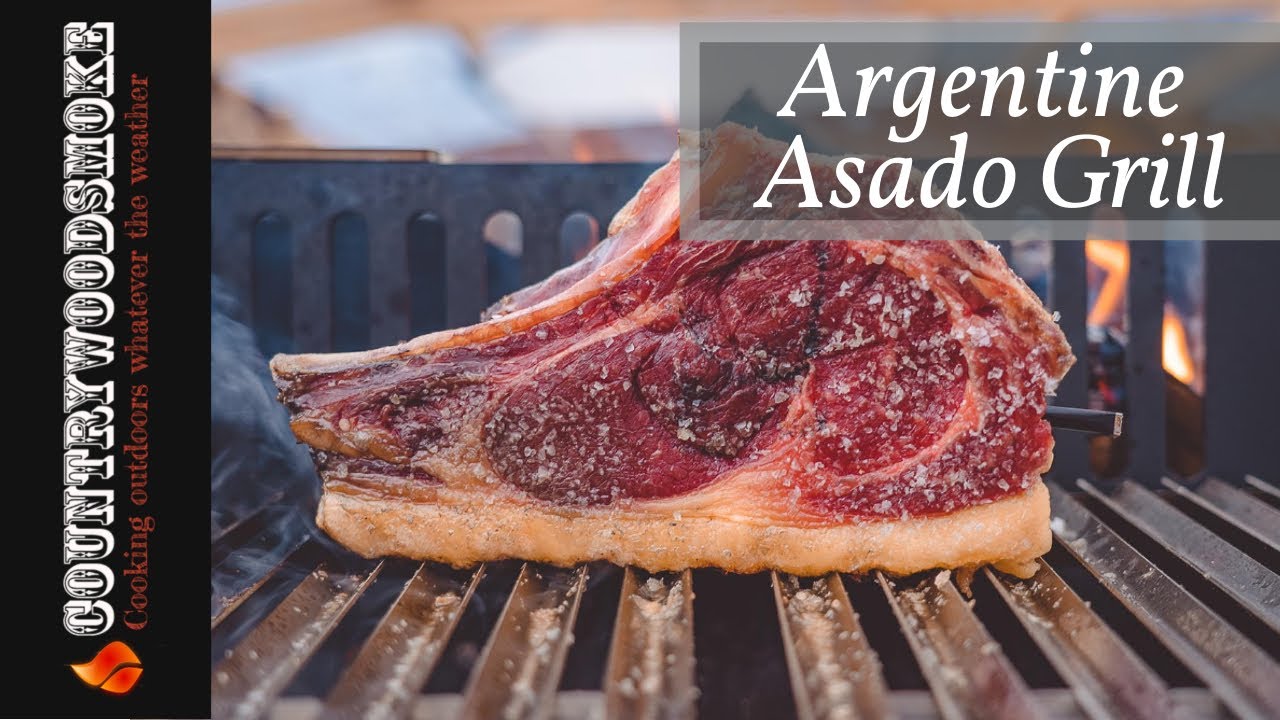This is a detailed image of a large, flapjack-like steak positioned prominently on a grill. The steak, with its moist, very red and luscious center, showcases a sizable bone at the top and is generously seasoned with coarse granules of salt. Dark grilling marks are visible on its surface, adding to its appealing presentation. The bottom part of the meat is distinguished by a thick, yellowish layer of fat. 

The grill beneath the steak emits rising smoke, contributing to the rustic ambiance. In the top right corner of the image, a semi-transparent gray text box bears the white inscription "Argentine asado grill," allowing the flames and the meat to be faintly visible through the text. On the left side of the image, a vertical black border contains white text in an old Western-style font that reads "Country Wood Smoke." Below this in smaller orange text is the phrase "Cooking outdoors whatever the weather," accompanied by a small flame symbol. The entire scene encapsulates an evocative essence of outdoor cooking and traditional barbecue experiences.